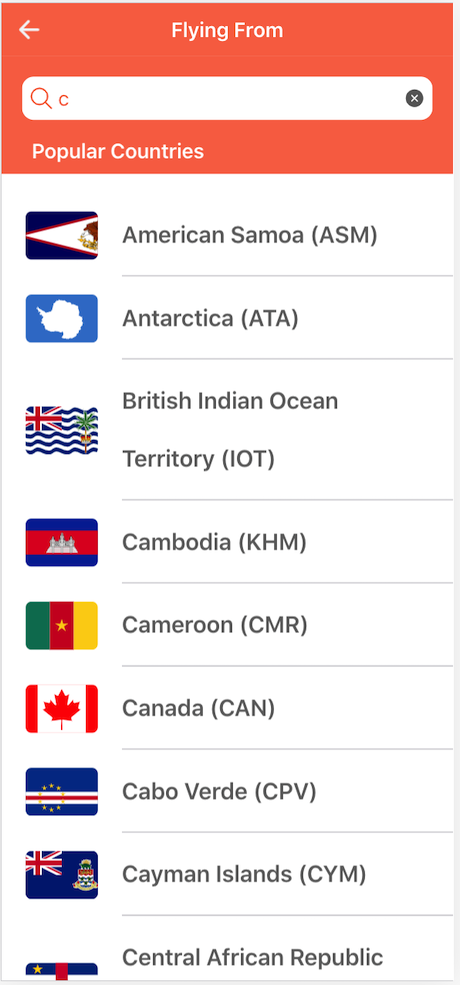The image is a screenshot from a website displaying a search interface for selecting countries. At the top, there is a banner in a melon color leaning more towards orange, featuring a white arrow pointing to the left. Centered on the banner is the text "Flying From," with both 'F's capitalized. Beneath the banner is a search bar that also shares the melon-orange hue, adorned with a magnifying glass icon followed by the letter 'C'.

Below the search bar, there's a white circular icon with an 'X' inside. Underneath this icon, the text "Popular Countries" is presented with both 'P' and 'C' capitalized. The section lists countries in alphabetical order, beginning with their respective flags.

The countries listed include:
1. American Samoa
2. Antarctica
3. British Indian Ocean Territory
4. Cambodia
5. Cameroon
6. Canada
7. Cabo Verde
8. Cayman Islands
9. Central African Republic (whose flag is partially cut off)

Each country is followed by its corresponding three-letter abbreviation in parentheses.